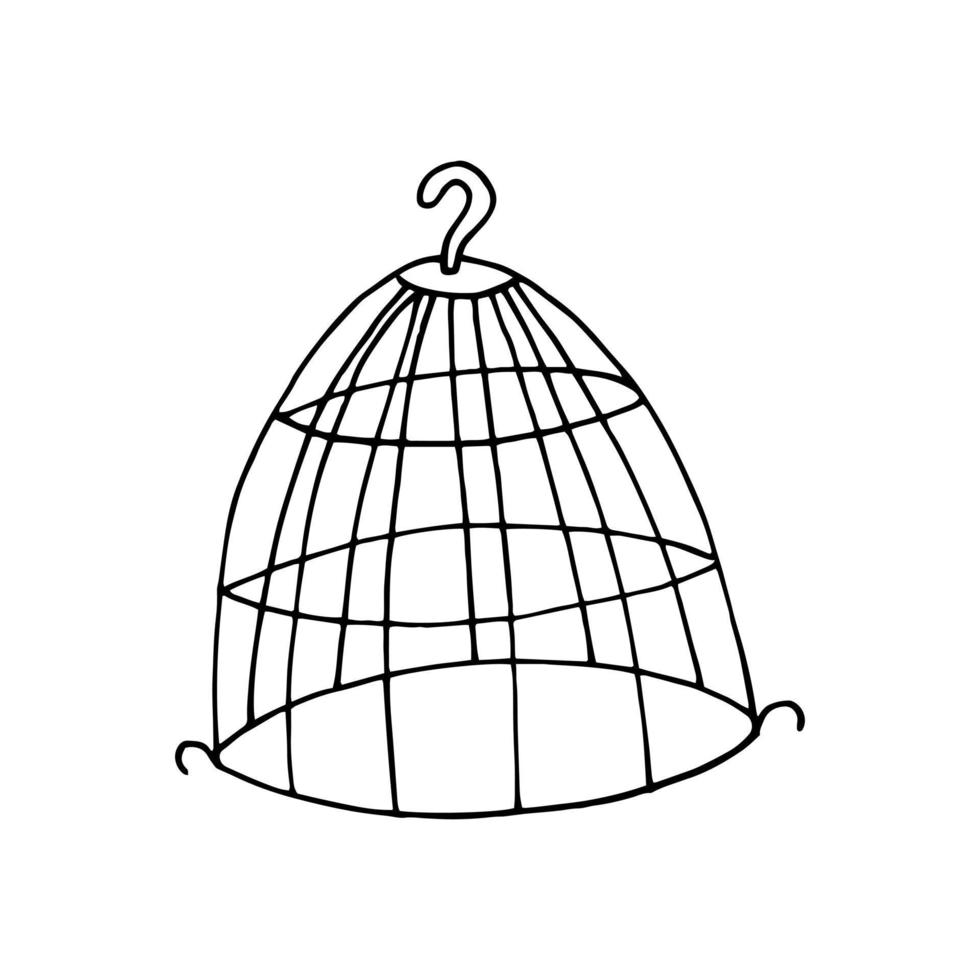The image is an intricate black and white illustration of the top part of a birdcage, rendered with whimsical, hand-drawn line art. The cage features a hook at the top, resembling a question mark, attached to a circular plate, suggesting it's designed to be hung either indoors or outdoors. The cage itself is designed like a rigid metallic net, characterized by its dark, uneven lines that add to its charming and academic aesthetic. Notably, the cage does not have a bottom, but includes two small hooks on either side near the bottom, indicating where a base could be attached. This detail hints that it's designed to be part of a complete structure, either for housing birds or fitting into another assembly such as a hoop skirt or mannequin component.